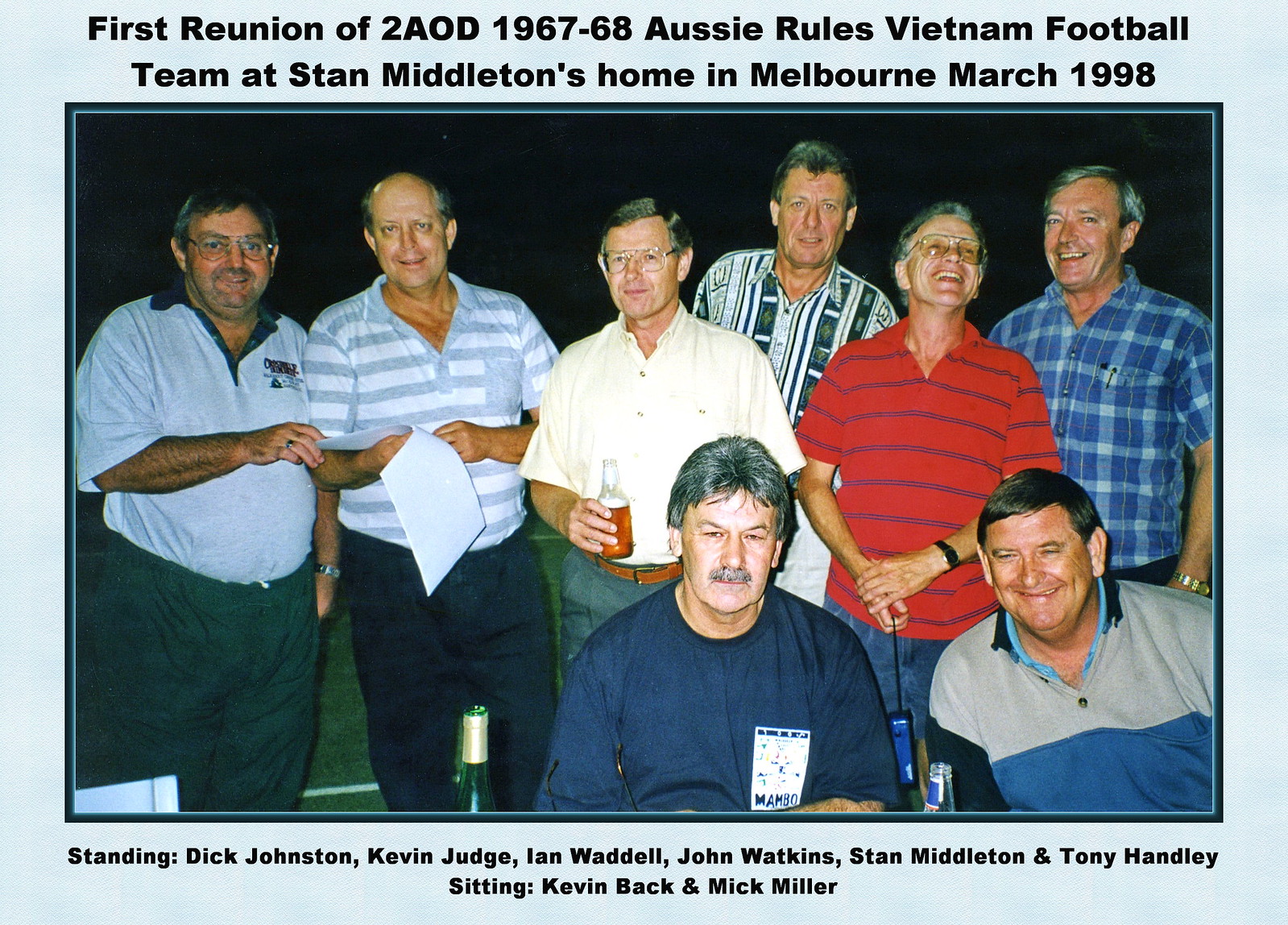In the photograph, a group of eight middle-aged men, ranging from approximately 40 to 70 years old, are posed in two rows for a picture. The back row, comprised of six men, features Dick Johnson, Kevin Judge, Ian Waddell, John Watkins, Stan Middleton, and Tony Handley. In the front row, seated, are Kevin Back and Mitch Miller. Most of the men are looking directly at the camera with cheerful expressions, some holding alcoholic beverages, papers, or other personal items. The photo is captured in color, showcasing their diverse attire in shades of red, blue, white, gray, and teal. Above and below the image, text reads: "First reunion of the 2AOD 1967-1968 All-Sea Rules Vietnam football team at Stan Middleton's home in Melbourne, March of 1998."